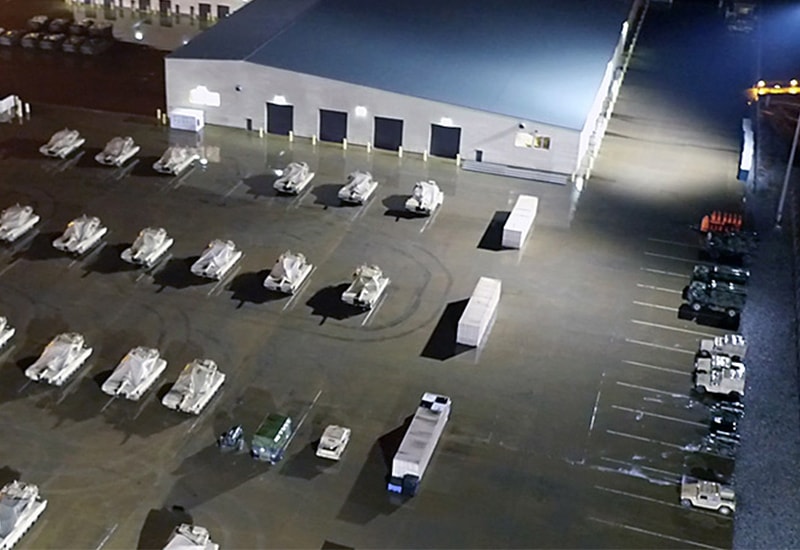This nighttime photograph captures a vast warehouse complex enveloped by an expansive parking lot and driveway. The white warehouse, standing prominently, features four dark-colored doors along its front facade. Its structure is topped with a medium blue, possibly metal roof that contrasts softly against the building's lighter exterior. 

On the right-hand side of the parking lot, several parking spaces are occupied by a variety of vehicles. Notably, there's a solitary car, followed by a few more vehicles, including white SUVs and some black vehicles, scattered across the lot. Additionally, the image reveals meticulously arranged rows of tanks, with four visible rows extending into the distance, further emphasizing the organized industrial nature of the scene.